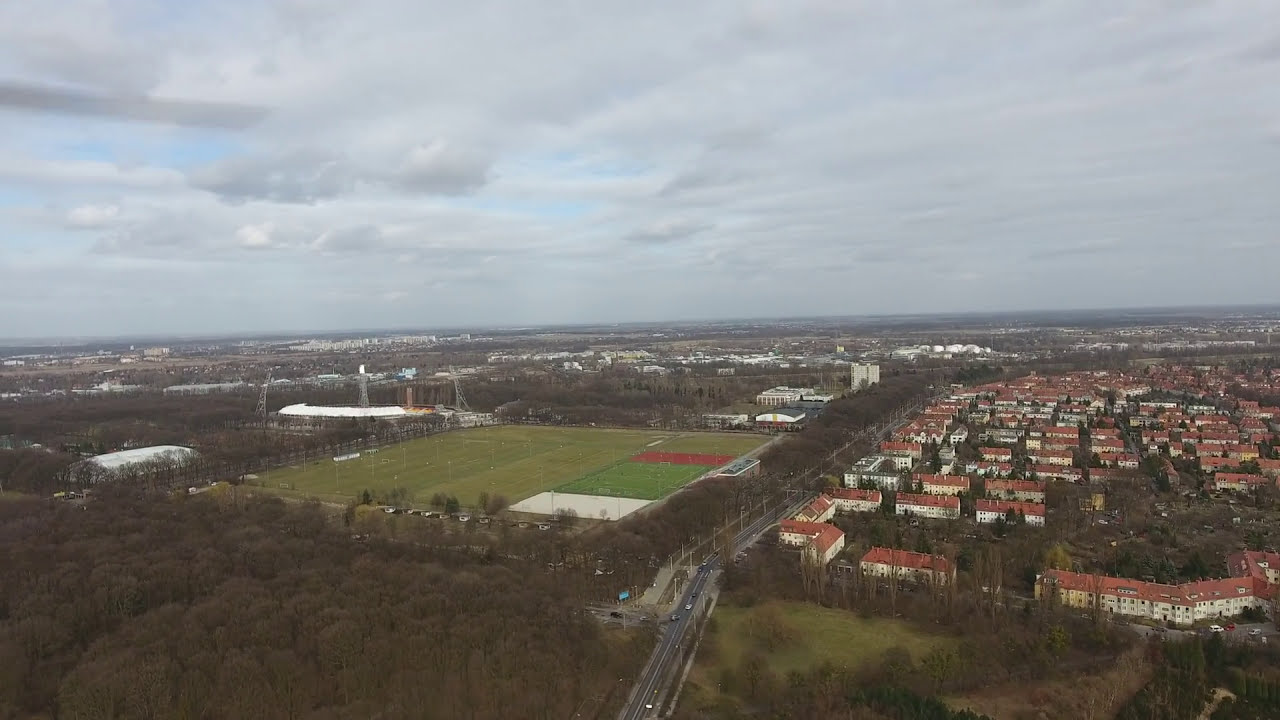This detailed aerial image captures a suburban landscape under a gray, overcast sky with hints of blue peeking through the clouds. The horizon line divides the image roughly in the middle. In the lower horizontal half, the left side features a large athletic field, possibly for football or soccer, bordered by a thick perimeter of trees and a dense thicket in the bottom left-hand corner. The right side of the image showcases a neighborhood with rows of white buildings topped with distinctive red roofs, suggesting either houses or apartments. A road runs towards the bottom center, populated with vehicles. The scene extends to other buildings in the distance, indicating the outskirts of a small city or suburb. The image is taken from a significant elevation, perhaps by a plane or drone, providing a comprehensive view of the landscape below.